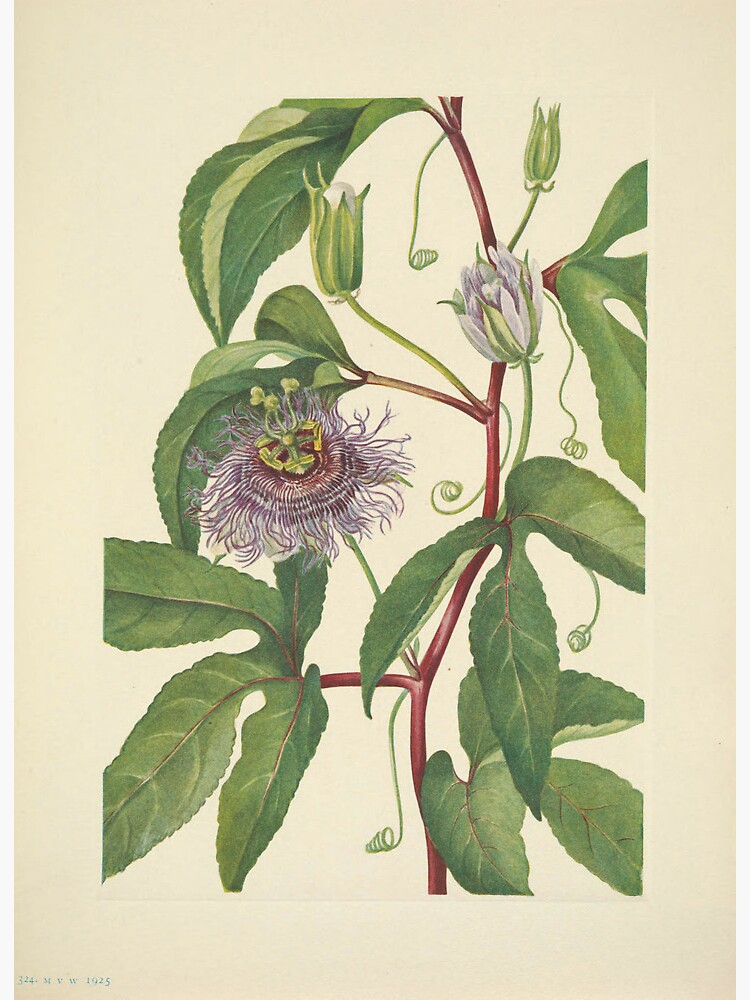This image is an intricate hand-drawn or painted artwork of a flowering plant set against an off-white, peachish-pink background. The plant features a reddish-brown stem that extends upwards through the center of the image and gently curves off to the side. There are several green leaves branching out from the stem, each with three smaller leaflets. On the right side of the stem, above the second set of leaves, a medium-sized purple flower is in full bloom, displaying green inner petals. Next to this flower, higher up, is a smaller bud that has yet to open. On the left side, a fully opened flower with hair-like purple extensions adds a pop of color. Above this, another stem branches out with additional green leaves, leading to a closed flower bud poised to bloom. Towards the top of the plant, another unopened bud is visible. The detailed depiction of the plant showcases an array of green leaves, reddish-brown stems, and varying stages of flowers, creating a visually striking composition.